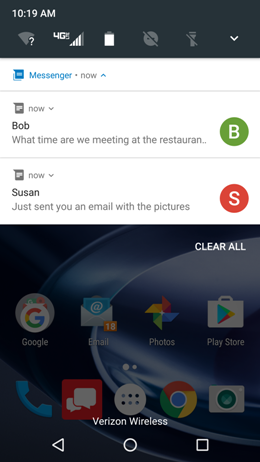In this detailed screenshot of a mobile device, the top left corner clearly displays the time, which is 10:19 AM. Adjacent to the time, vital status icons are visible, including the Wi-Fi signal strength, the 4G LTE connectivity symbol, and the battery level indicator. Notably, the "Do Not Disturb" mode is active.

Foregrounding the screen are several notifications: one from Bob inquiring, "What time are we meeting at the restaurant?" and another from Susan stating, "I just sent you an email with the pictures." The device's home screen background showcases various app icons, such as Google, Email, Photos, Play Store, the Phone Dialer app, and another instance of the Google app. The meticulous arrangement and clarity of the icons provide a comprehensive view of the device's configuration at a glance.